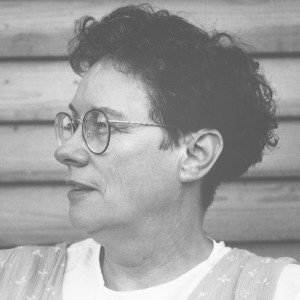This black and white photograph captures a close-up profile of an older woman, likely in her 50s, facing towards the left. Her short, dark hair—possibly dark brown—frames her face, and she wears distinctive circular wire-rimmed prescription glasses. Her facial features include a slightly pointy nose, and though only her left eye is clearly visible, the right eye is hinted at due to the slight tilt of her head.

She is clad in a white shirt, layered beneath what appears to be a darker-colored vest or the bodice of an old-fashioned dress, possibly with a floral pattern. The backdrop consists of horizontal wooden slats, suggesting the wall of a building, though the exact details are elusive due to the extreme close-up nature of the photograph. The composition and attire hint at an era gone by, capturing a moment in the life of a woman whose attire suggests she has possibly led a challenging life.